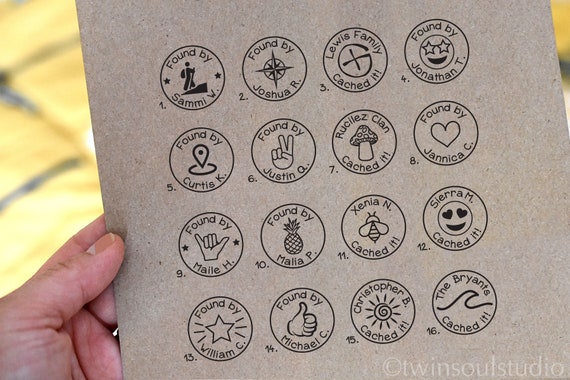This full-color, square photograph taken indoors with artificial light, displays a human hand – specifically the left hand of a Caucasian person, holding a dark brown cardboard sheet. There are 16 circular stamps arranged in a grid with four rows of four, numbered 1 through 16. Each circle contains black text and simple black line drawings. The text within these circles includes phrases like "Found by Sammy," "Found by Joshua R.," "Found by Jessica C.," and "Caught by the Lewis Family," often accompanied by symbols such as stars or stick figures. The background of the image is a plain, yellowish color, allowing the brown paper to dominate the composition. A watermark in the lower right corner identifies the creator as Twin Souls Studio. The stamps, resembling postmarks but lacking the typical information, suggest they might be related to a game or scavenger hunt.